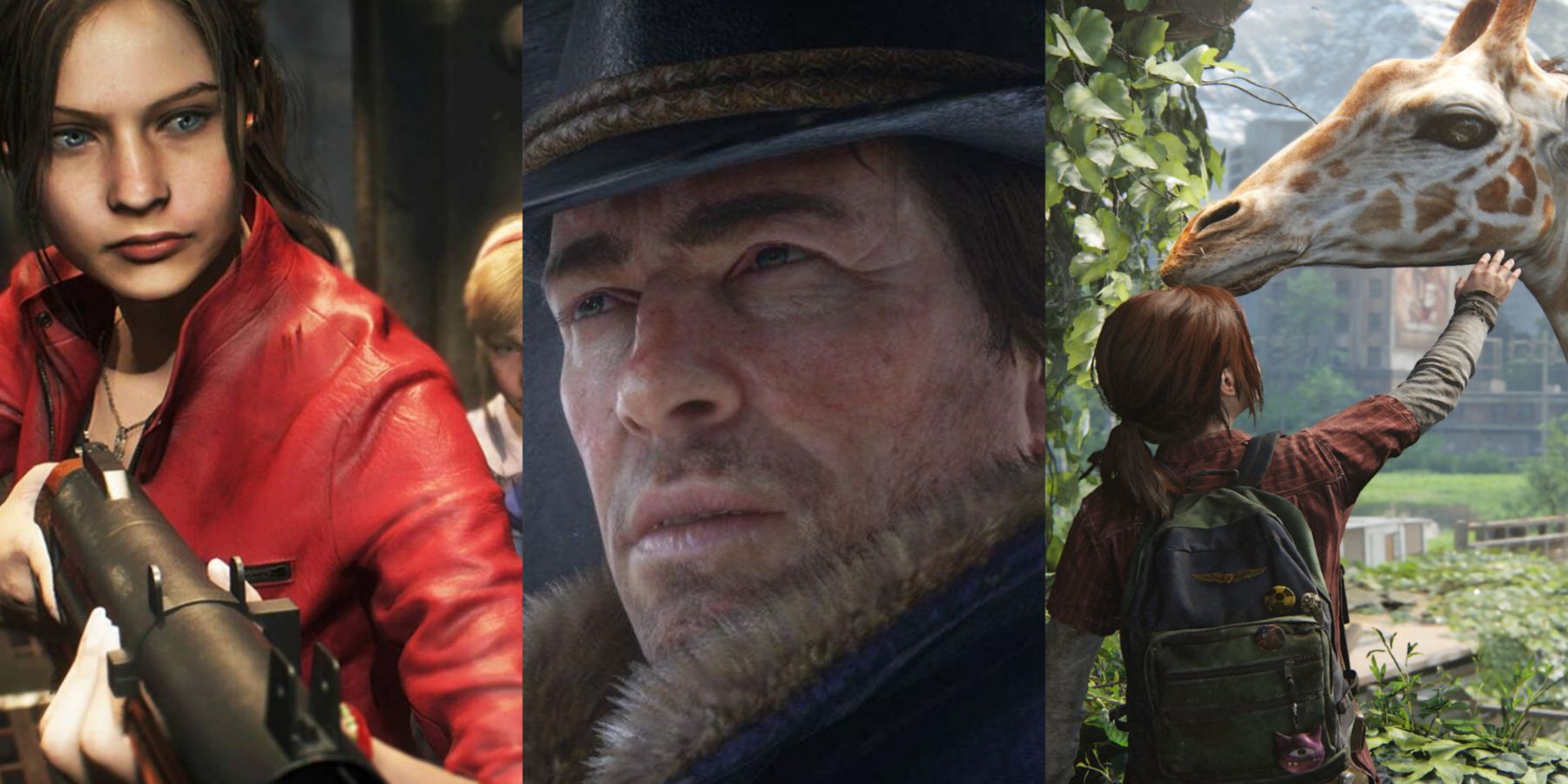This image consists of three side-by-side AI-generated pictures designed to mimic realistic human portraits. Each segment portrays a distinct character and setting. On the left, there is a close-up of a woman with dark brown hair and striking bright blue eyes. She is dressed in a red leather jacket and a necklace, holding a gun pointed at someone with an intense, serious expression. The middle image features a grizzled man with a rugged appearance, wearing a cowboy-style black hat and a coat with a fur collar. His serious demeanor also suggests tension. The rightmost picture depicts a young girl in a red shirt and backpack, viewed from behind, as she reaches up to pet the face of a giraffe. The scene includes greenery, indicating it is outdoors, and the giraffe's face is visible, munching on leaves. The combined effect of these AI-rendered images creates a vivid, dramatic tableau reminiscent of a video game or cinematic sequence.